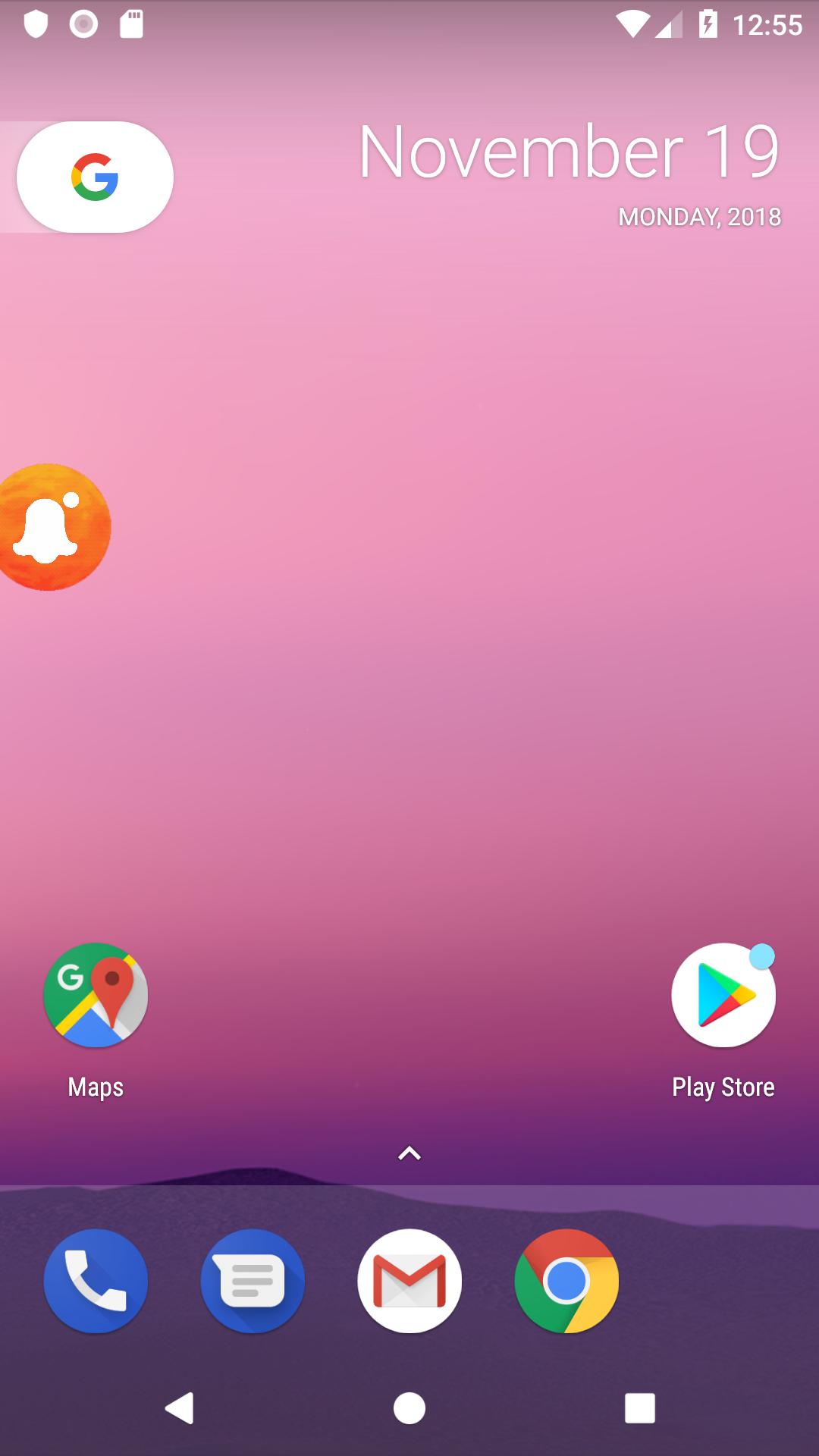The image is a screenshot of a smartphone's home screen, showcasing a minimalistic arrangement of apps against a serene background. At the top right, the time is displayed as 12:55, with the battery icon indicating that the phone is nearly fully charged and currently plugged in, as evidenced by the lightning bolt symbol. Directly beneath the time, the date reads "Monday, November 19, 2018."

On the top left of the screen is the Google app icon, recognizable as the browser. Below that, roughly in the middle left, there is an unusual orange circle icon, which appears to be for Snapchat, though it differs from the app's typical logo. In the bottom left corner is the Google Maps app, while the Google Play Store icon occupies the bottom right corner.

The dock at the bottom of the screen features four pinned apps from left to right: the phone app, text messaging app, Gmail, and Google Chrome, indicating that Google Chrome is their primary browser. The background image is a tranquil sunset scene, with shades of pink and purple in a foggy sky, reflecting over a large body of water with islands in the distance.